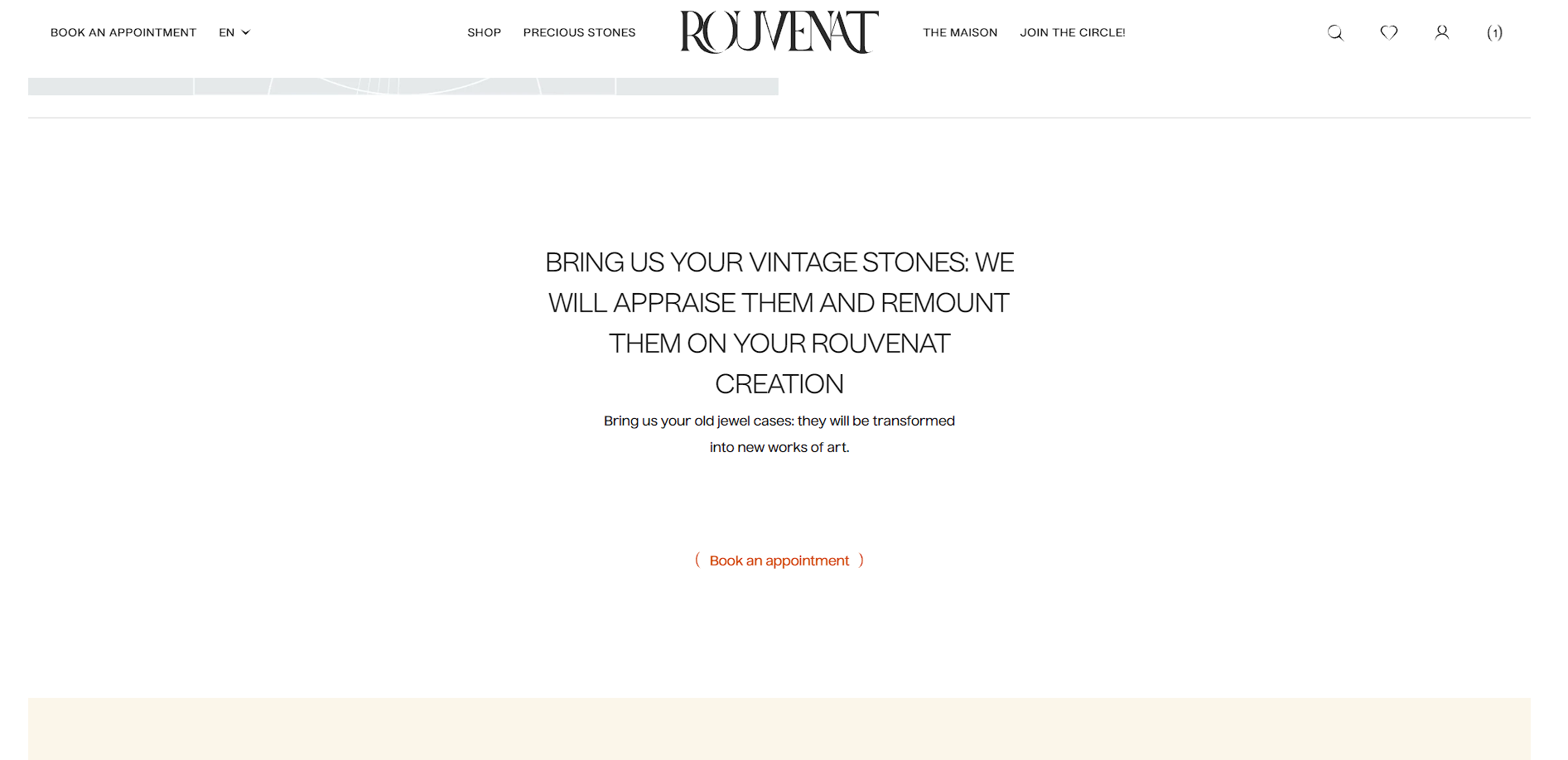The image features a predominantly white background with a variety of elements arranged across it. At the top, there is a small section containing the option to "Book an Appointment,” which includes an active drop-down menu with selections such as "Shop" and "Precious Stones." Below this, the name "Revenant" is prominently displayed, followed by "The Madison" and an option to "Join the Group." To the right, there are several small icons. A heavy blue line runs horizontally, accompanied by a smaller blue line beneath it. The central portion of the image invites viewers to "Bring us your vintage stones; we will appraise them and remount them on your Revenant creation. Bring us your old jewel cases, they will be transformed." There is also a very small, unreadable line below this text. In red, within parentheses, is the phrase "Make an appointment." The bottom of the image features a light-colored red box.